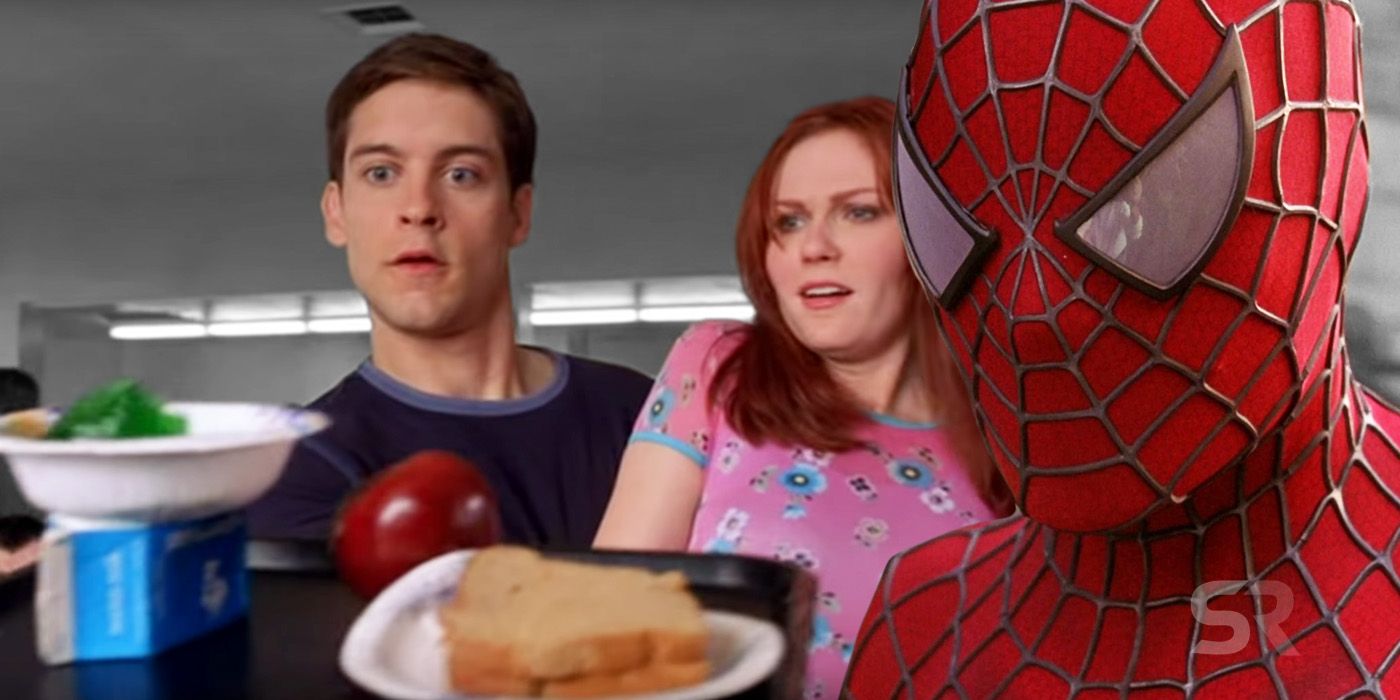In this landscape-oriented image with a dramatically rectangular layout, Spider-Man's head and a portion of his chest dominate the right side. The iconic red mask features a charcoal-colored web pattern extending from between his eyes across his face and down his body. To the left of Spider-Man, actors Tobey Maguire and Kirsten Dunst, both Caucasian, capture attention. Tobey, with brown hair and a black shirt, stands close to Kirsten, who sports red hair and a pink and yellow floral shirt. Both actors appear to be gazing downward with an alarmed expression. In front of them, occupying the lower left-hand corner, a black tray holds a white paper plate with a sandwich, a red apple, a blue milk carton, and a white paper bowl containing lettuce. Depicted against the backdrop of a white ceiling with lights, the combined elements of this image suggest a stylized, representational photograph with special effects, making it appear as though the characters are intently focused on the seemingly mundane cafeteria tray below them.